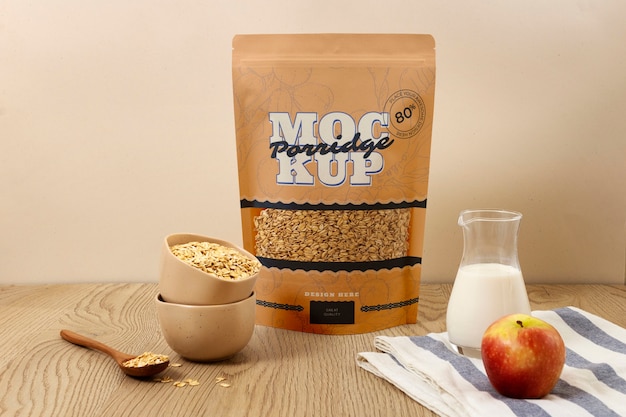In a cozy breakfast scene set against a yellow-tan wall, a wooden table with pronounced vertical grain hosts a selection of morning staples. Central to the image is a lightly orange packaging of porridge branded "Mock K.U.P. porridge" with white block letters and black script. A clear cellophane window in the package reveals the porridge inside, accentuated by small black lines. On its left, two stacked bowls showcase the porridge, the top bowl partially served with a wooden spoon resting inside, and some porridge flakes spilling onto the table. To the right of the package, a see-through glass pitcher of milk and a vivid red apple rest on a white and gray striped towel. The scene is a blend of warm and inviting tones, capturing the simple yet satisfying ambiance of a breakfast setting.